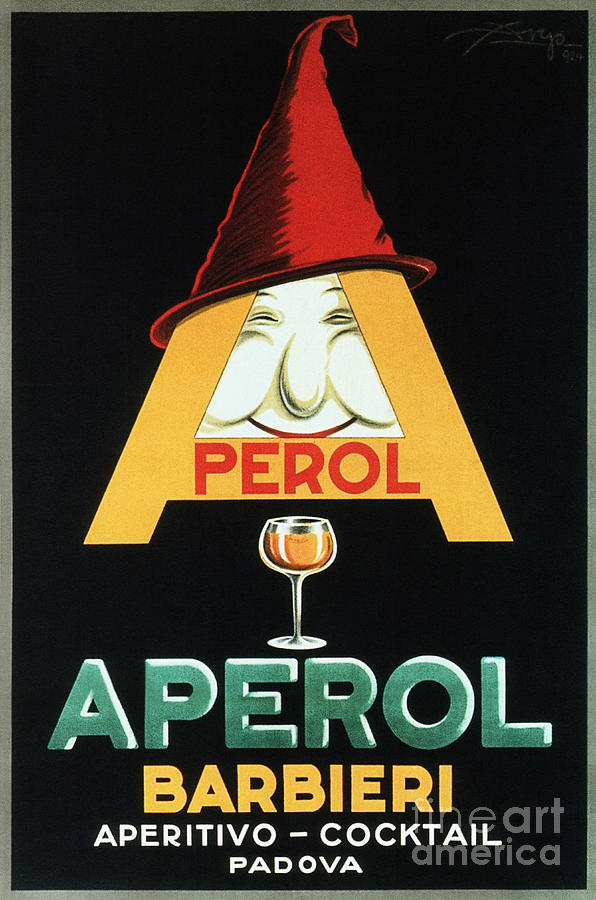This is an advertisement that features a striking design set against a jet-black background. Central to the image is a gigantic, yellow letter "A" adorned with a dark red witch's hat, identified by its curled and rolled-up tip. The middle of the "A" showcases a mischievously smiling, long-nosed face with chubby cheeks that adds a touch of whimsy or eeriness, depending on your perspective. Written across the letter "A" is the word "PEROL," and just below it, there is a Y-shaped wine glass containing a yellowish-orange beverage. Further down, vibrant green lettering spells "Aperol," followed by the gold word "Barbary," and ending with the phrase "Aperitivo Cocktail Padova" in small white letters. The poster also mentions "Great America" subtly on the right-hand side, tying the advertisement together with an air of international sophistication.